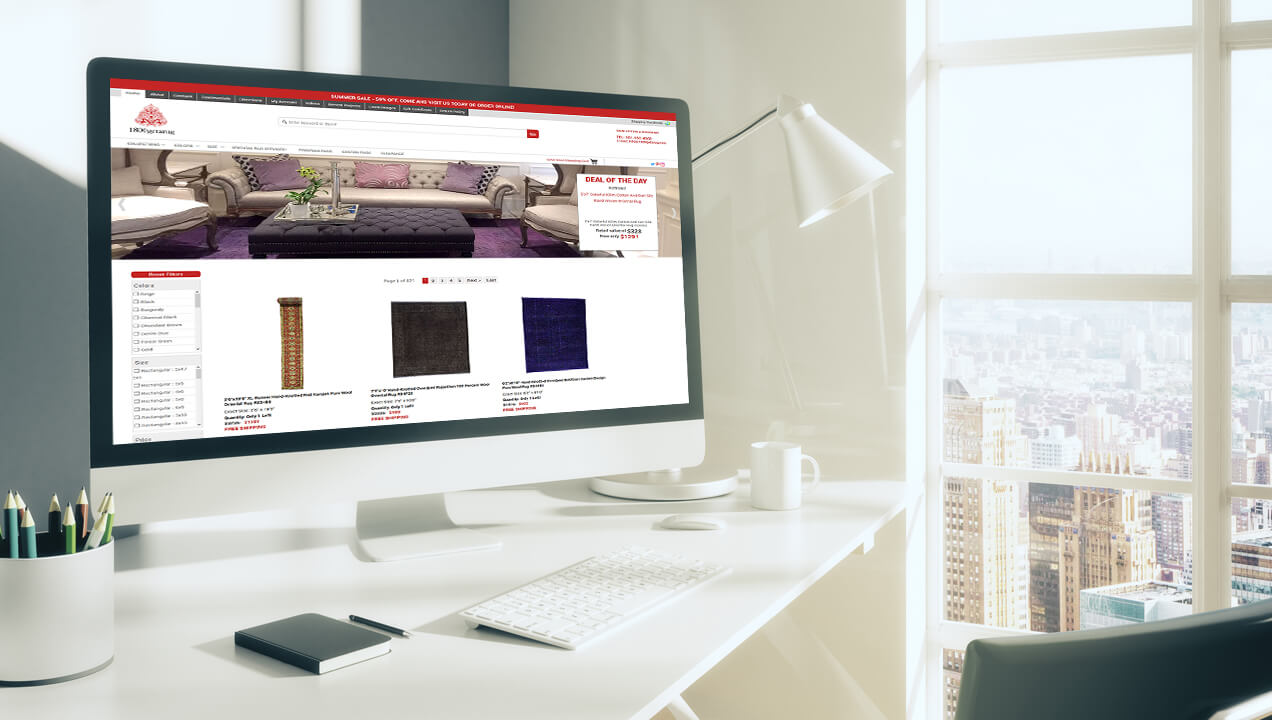A pristine and organized home office is featured in this photograph. In the background, a large window offers a picturesque view of a bustling cityscape. The focal point, a sleek white desk, is adorned with several minimalist accessories. A modern white lamp sits neatly towards the back, casting a soft glow over the workspace. In front of the lamp, a classic white mug adds a touch of simplicity to the scene. Prominently positioned in the foreground is a white pencil holder, next to a sophisticated black notebook paired with a matching black pen.

A white keyboard, presumably used for a Mac, hints at the technology that powers this workspace. Dominating the desk is a larger iMac screen. On the screen, an online shopping site is displayed, highlighting the "Deal of the Day." Various photographs of rugs, likely on discount, spread across the screen, indicating someone might be in the midst of redecorating.

Completing the setting, a comfortable black desk chair is pulled out, ready for the next user to settle in. The overall look is one of modern elegance, efficiency, and understated style.